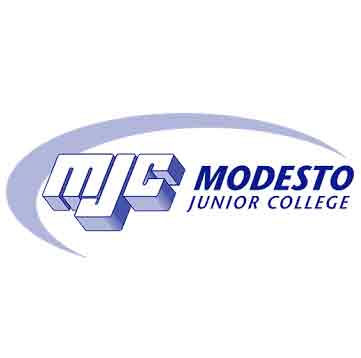This image features the detailed logo of Modesto Junior College. The logo is set against a white background, dominated by a blue and white color scheme. The most prominent element is the large, three-dimensional block letters 'MJC', which appear in white with blue-shaded sides to enhance their 3D appearance. Surrounding the text is a light blue swoosh that begins at the lower left, curves gracefully over the top, and finishes towards the right of the text. To the right of the MJC initials, the word "Modesto" is displayed in bold, dark blue letters that stand out prominently. Beneath "Modesto" are the words "Junior College" in a thinner, dark blue font, making it clearly readable but less dominant than "Modesto". The overall design integrates a moon-like crescent shape that visually connects the text elements, providing a cohesive and dynamic look.